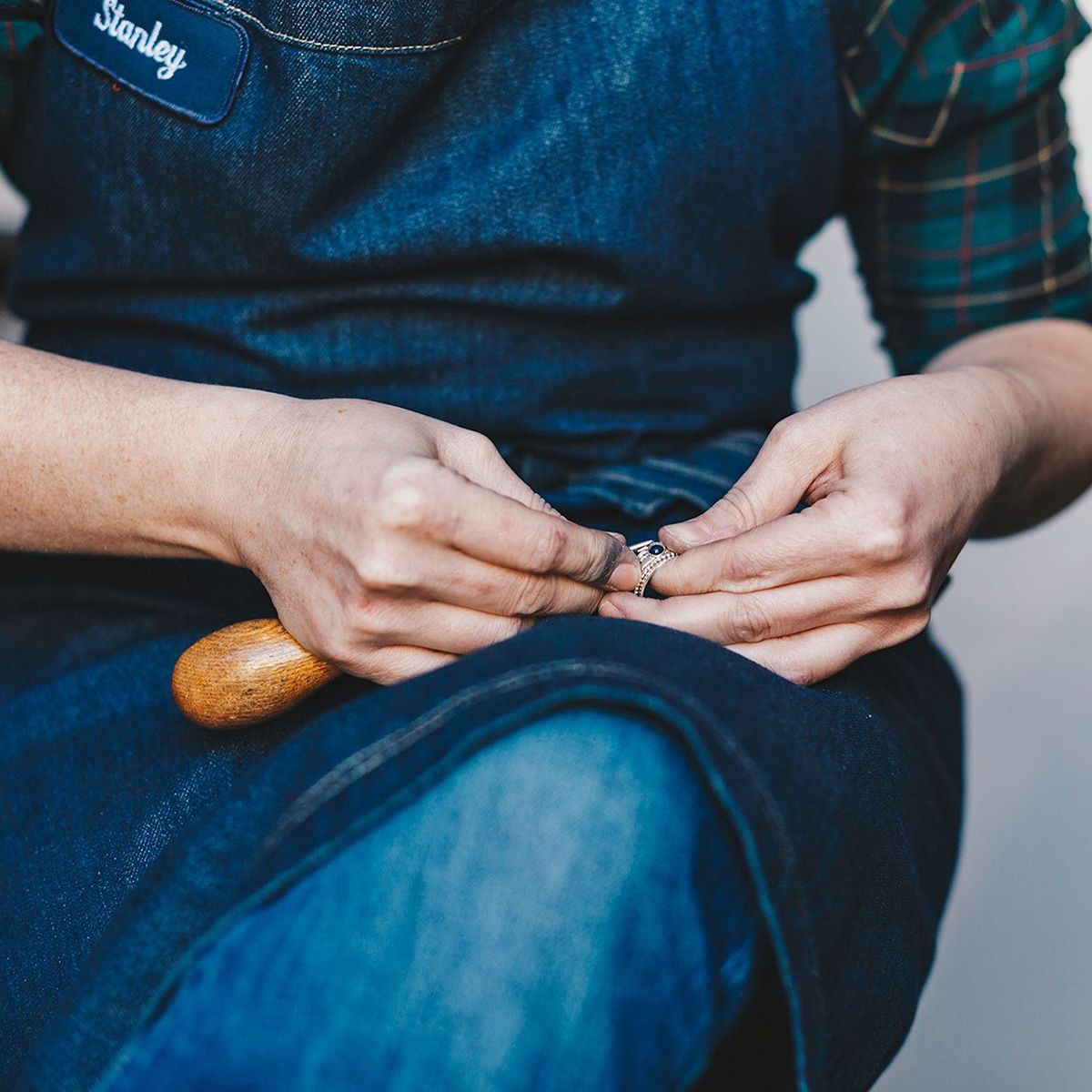In the image, a craftsman named Stanley, identifiable by the name tag on his denim apron, is meticulously working on a ring. Stanley is dressed in blue jeans and a plaid shirt with the sleeves rolled up, exposing part of his arm. His hands are prominently featured, with the left hand holding a ring and the right hand grasping a wooden-handled tool, possibly for setting a stone. The ring, which is either gold or silver with a distinctive design, features a dark jewel embedded in the center. The photograph is carefully composed to focus on Stanley's precise handwork, with his left leg serving as a steadying surface and both his jeans and apron blending into the background. The scene is intimate, capturing the essence of manual craftsmanship in a blurred, yet detailed, workspace.